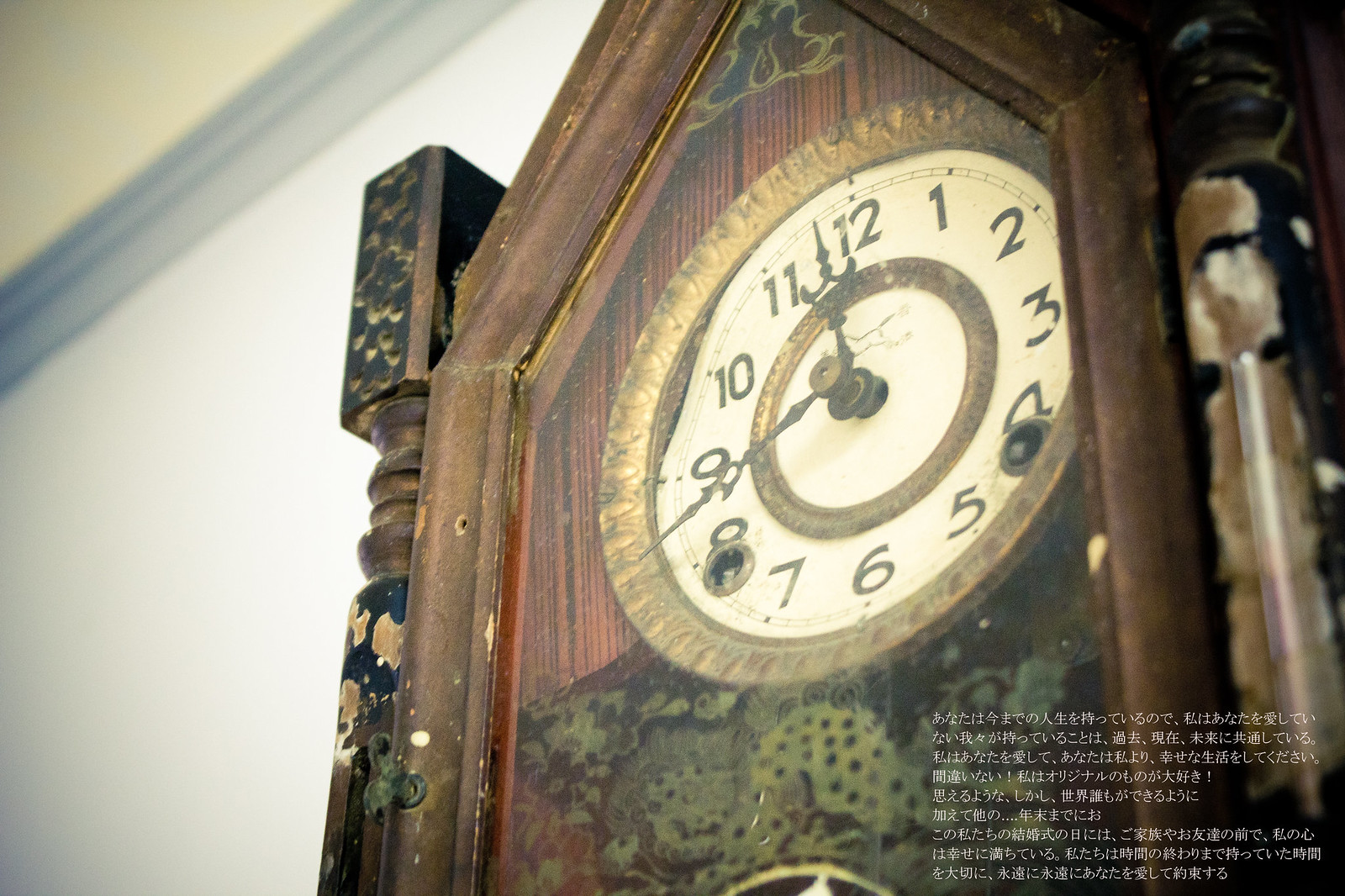This detailed caption portrays an image of an old, grandfather-style wall clock:

The image depicts a vintage wall clock reminiscent of a grandfather clock. The clock is housed in a wooden frame that shows signs of age and wear, with visible damage and a well-worn texture. The clock face is white with two ornate gold trims: one encircling the outer edge and a second, smaller circle just inside the numbers. The numbers, of course, range from 1 to 12 and are marked in a traditional style. The clock's hands are made of black metal, featuring intricate, decorative designs. The time displayed is approximately 20 minutes to 12. Below the clock face, there is a section highlighted with a green hue, appearing to be painted directly onto the clock. On the far right at the bottom, there is some text inscribed in white, which appears to be in an Asian script.